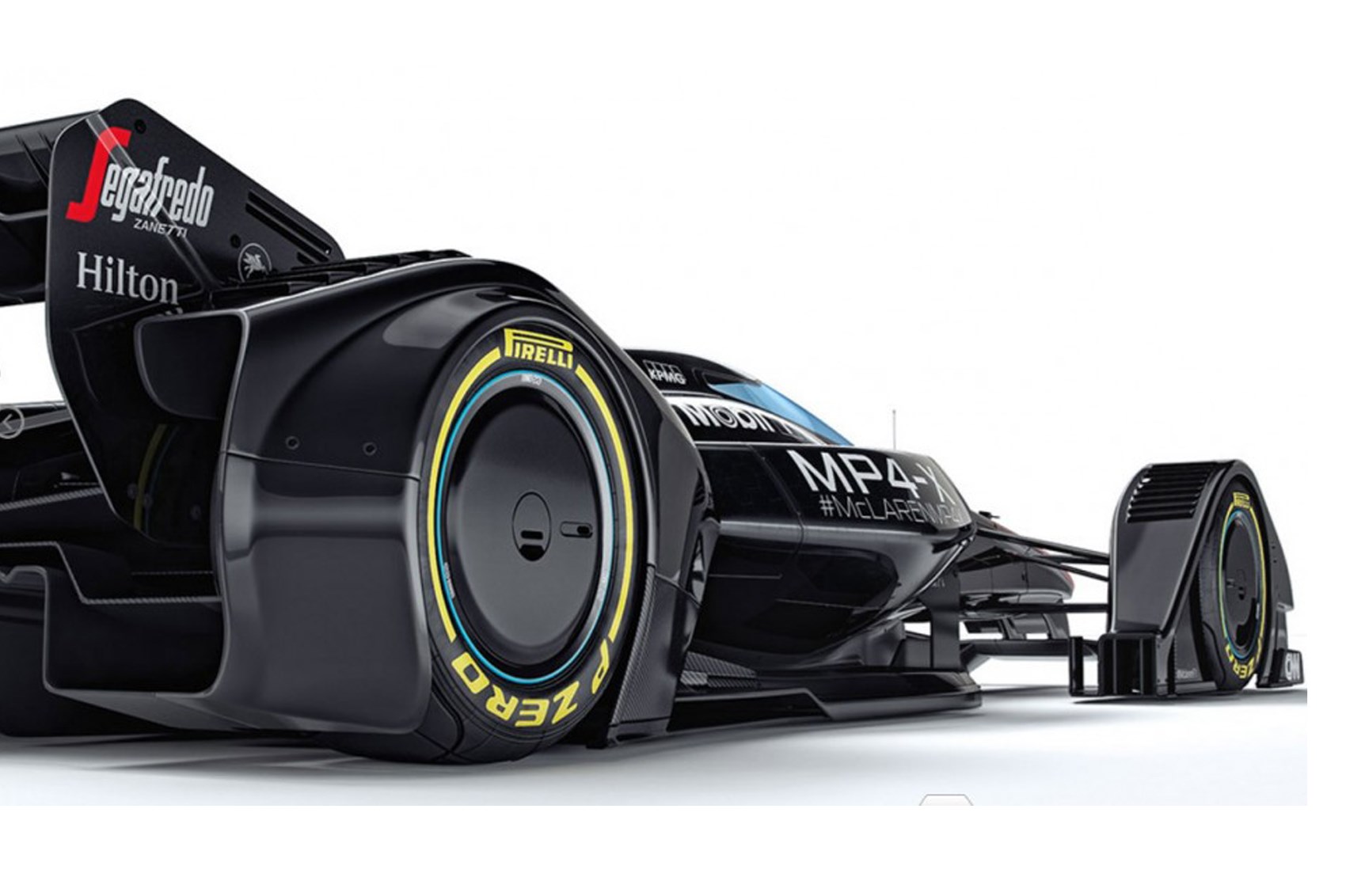The image showcases a sleek, black Formula One race car set against a pristine white background. Captured from a semi-profile view, as if standing behind the front right wheel, the car's tail end is positioned to the left side of the image. The race car's low-slung body lies almost flat against the white floor, a hallmark of high-performance design. Distinct branding and logos adorn the car, including "Segafredo Zanetti," "Hilton," and "Mobil," with "MP4-X" and "#McLaren" emblazoned on its streamlined surface. The wheels feature striking yellow trims marked "Pirelli" and "P0." The vehicle's front wheels are connected to the car body by visible black rods, enhancing its high-tech aesthetic. The car is very shiny, with gray wheels and additional colored trimmings in yellow, blue, and red.